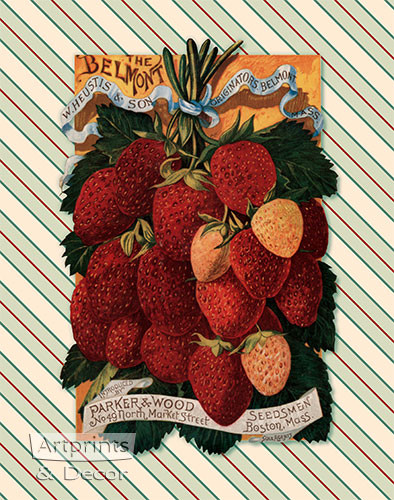This advertisement poster features a vintage illustration of a seed packet against a patterned background of angled stripes in olive green, dark green, beige, red, and teal. At its core, the image prominently displays a cluster of approximately 15 strawberries, ranging from dark red to light pink, suggesting varying ripeness. The strawberries are tied together by blue and white ribbons. The upper ribbon, in blue, reads "Houstis and Son, Originators Belmont, Mass," indicating the Belmont variety of strawberries from Belmont, Massachusetts. Below, a white banner states "Parker and Wood, Seedsmen 49 North Market Street, Boston, Mass." The background of the illustration is orange, with "The Belmont" inscribed in black text at the top left. To the right of the painting, there is additional text such as "art prints" in a white banner, and "decor," faded but still discernible. The combination of detailed artwork and historic text suggests it's possibly a reproduction of a classic seed packet design. The entire poster merges a nostalgic advertisement style with modern decorative elements, making it a unique piece of art.